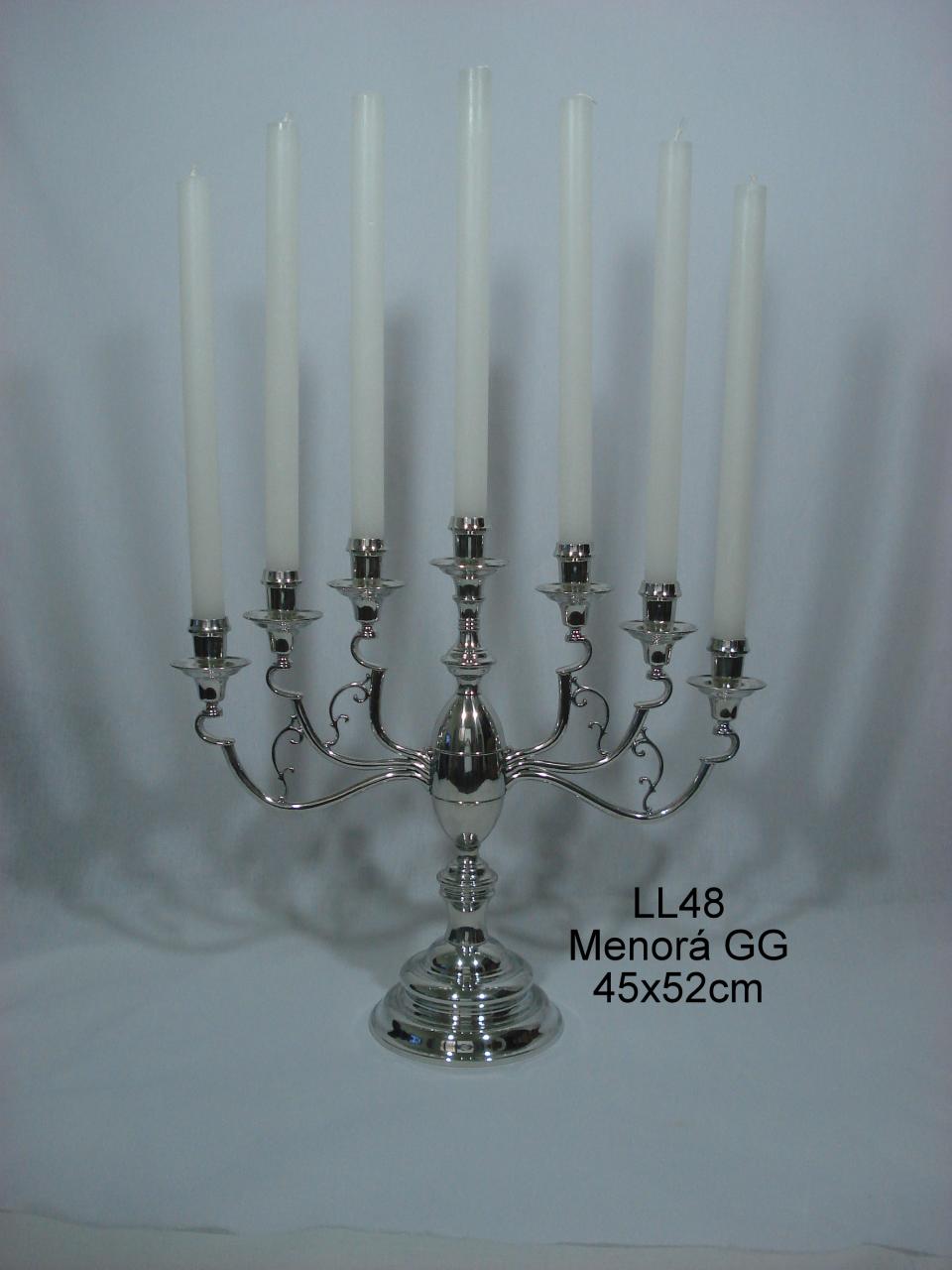The photograph depicts a highly polished, shiny silver menorah, also known as a candelabra, with seven ornate candlestick holders. Each holder accommodates a long, narrow, unlit white candle. The menorah is crafted in an intricate and decorative style, featuring curlicues and a central body that branches out, forming elegant, backward C-shaped arms that hold the candles. The background is a solid, medium gray that casts a pleasing shadow of the menorah, enhancing its visual appeal. To the right of the menorah, black text reads "LL48 Menorah GG 45 x 52 centimeters."